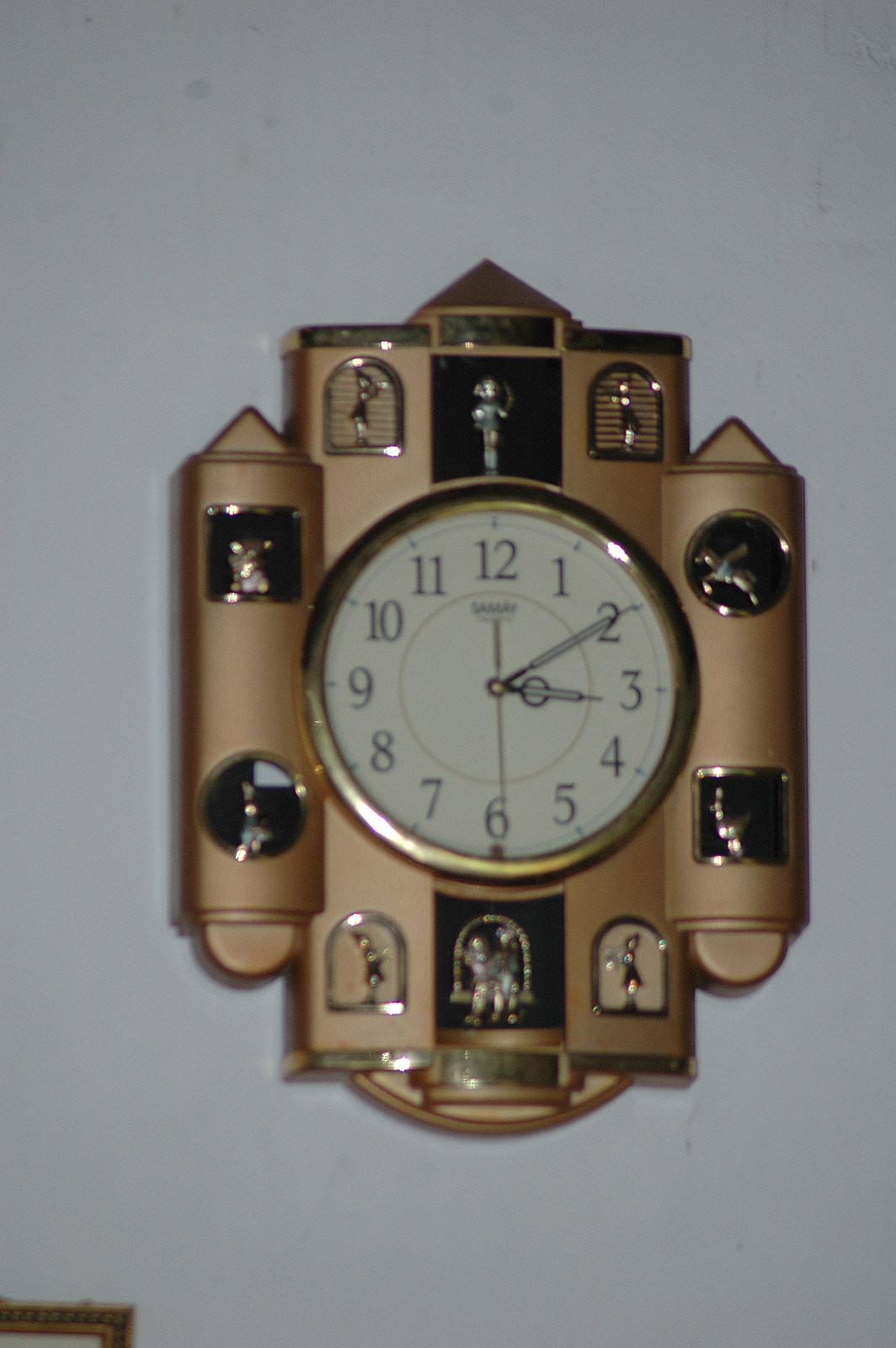A stately, decorative clock designed in the shape of a castle hangs prominently on a plain white wall. The distinctive bronze structure features intricate cutouts, each housing miniature golden statues that resemble dancers frozen in mid-pose. These cutouts, varying in shape from squares to circles and half-ovals with flat bottoms, encircle the clock's face, adding to its ornate appearance. The clock's face is white, punctuated by golden details that lend it an air of elegance. In the bottom left-hand corner of the frame, the edge of a photo frame peeks into view, suggesting the presence of other personal touches in the room.